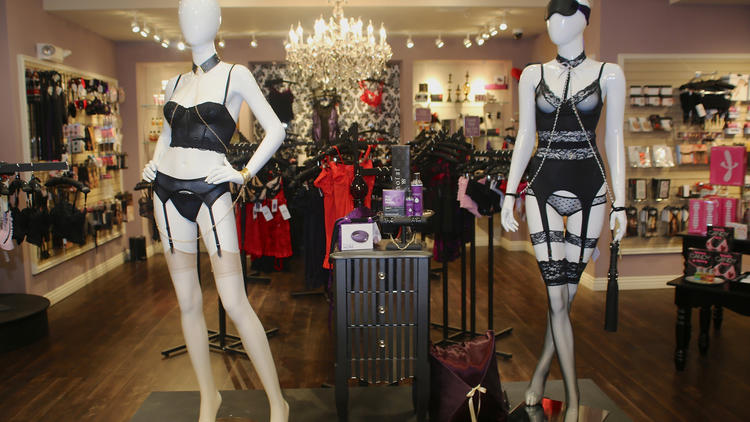This is a detailed photograph from an adult lingerie store. The focal point of the image features two white mannequins prominently displayed in black lingerie. The mannequin on the left is bald and adorned with a necklace, a brassiere, underwear, a garter belt, and flesh-colored tights. The right mannequin wears a sleep mask partially covering its face, a neck brace with chains attached to wrist bracelets, black garter belt underwear, and sheer black stockings. Both mannequins stand near a table with indistinct purple items. In the background, shelves and racks display various adult toys, lingerie, and clothing items, including notable red and black articles of clothing. Some pink boxes with the silhouettes of sex toys are visible on the right. The scene is illuminated by a chandelier hanging from the ceiling, giving the space a high-end boutique ambiance. The overall decor includes a wooden floor, gray walls, and spotlights that accentuate the merchandise.